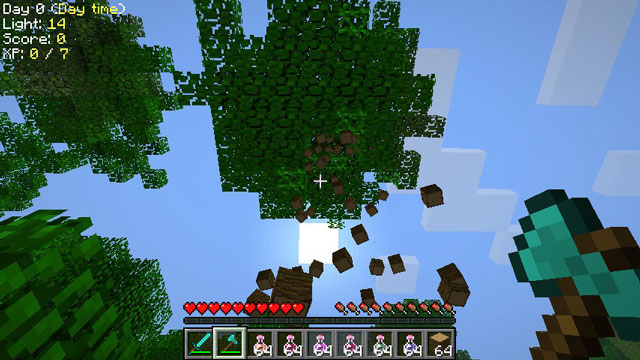This image appears to be a screenshot from the popular game Minecraft. Dominating the right-hand corner are distinguishable green, brown, and black blocks, hallmark textures of the game's voxel-based world. The background showcases a vibrant blue sky, while the left and upper left-hand corners, as well as the center, are adorned with lush foliage.

In the upper portion of the screen, several blocks are seen descending, indicative of active gameplay. At the bottom of the screen, there's a HUD (Heads-Up Display) showing a row of hearts, likely representing the player’s health, and a row of icons resembling goblets, which might denote experience levels or potions.

Further below, there are icons of a sword, an axe, and other items, each marked with the number 64, suggesting a maximum stack of these items in the player's inventory. The left-hand corner of the screen displays vital in-game information: "Day 0," "Light: 14," "Score: 0," and "XP: 0/7," reflecting the player’s current conditions and statistics in the game world.